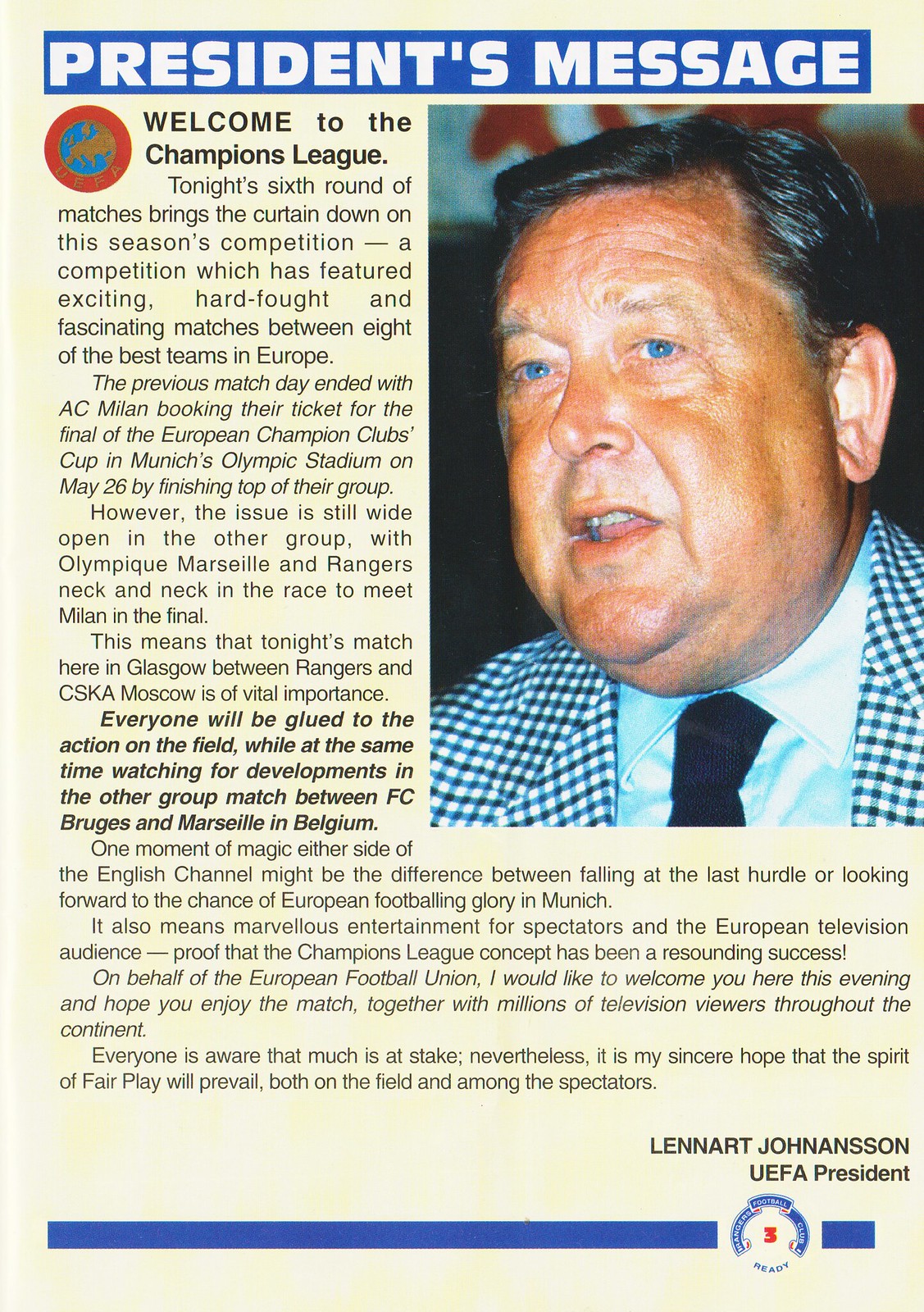This image showcases a flyer or pamphlet, potentially from a magazine, featuring a message from the president of a football league. The flyer has a predominantly pink background with a horizontal blue bar at the top, displaying "PRESIDENT'S MESSAGE" in capital white letters. To the right underneath this bar, there's a picture of Lennart Johansson, the UEFA president, who is an elder gentleman with dark hair and blue eyes. He is depicted wearing a checkered suit jacket, a blue tie, and a white shirt.

The text begins with a warm welcome to the Champions League, emphasizing the thrilling nature of the season's sixth round of matches, which bring to a close this year's competition. It highlights the participation of eight of Europe's top football teams, and mentions the excitement surrounding AC Milan advancing to the final of the European Champion Clubs Cup at Munich's Olympic Stadium on May 26th. Additionally, the flyer references other prominent teams, including the Rangers and Olympique Marseille, noting their involvement in matches played in Glasgow.

The president’s message is described in detailed paragraphs spanning the flyer, concluding with Leonard Johansson's name and title, "UEFA President," positioned above the UEFA league logo and a blue line at the bottom. The main colors used throughout the flyer are blue, yellow, black, and white, creating a visually cohesive and professional presentation.